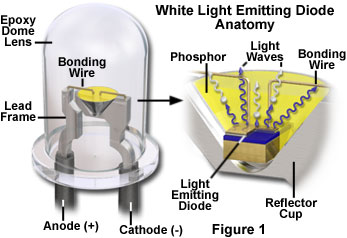The image is a detailed diagram titled "White Light Emitting Diode Anatomy," set against a white background. Central to the illustration is an LED with a glass-like epoxy dome that houses the core components responsible for light emission. The diagram highlights the phosphor layer, depicted as a yellow triangle with blue and white squiggly lines, indicating where the conversion of light occurs. Key parts labeled include the bonding wire, lead frame, anode (positive), and cathode (negative). An inset image offers an enlarged view of the central section, reinforcing the importance of the structure labeled as the light-emitting diode. Additional annotations identify the reflector cup and the epoxy dome lens, which protect and enhance the light output. The diagram is comprehensive, providing a clear breakdown of each component's role in the functioning of a white light LED.